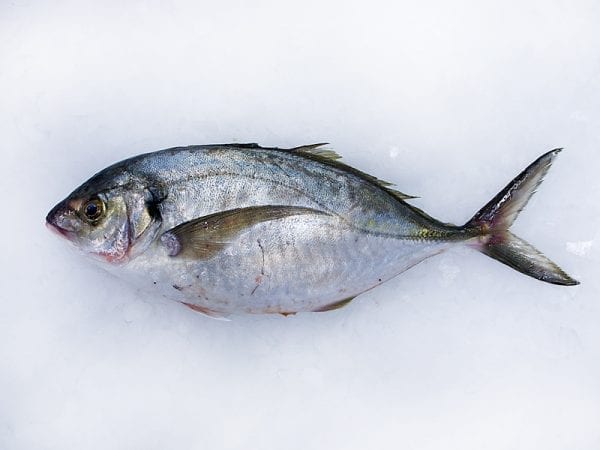The image depicts a dead, silvery fish lying on an icy white surface, with its body angled to the left. The fish’s singular visible eye is open, revealing a black pupil with brown edges, while its closed mouth shows a hint of red. Its wide, oval-shaped body, reminiscent of a football, extends to the right where a grayish-white, V-shaped tail points both up and down. The fish’s silver scales shimmer with hues of gold and yellow, adding to its reflective appearance. Notably, a brown dorsal fin can be seen extending from its back. Additionally, faint fuzz or fur-like material traces the outline of its belly, contributing a delicate texture to the overall image. The stark white background highlights the fish's muted colors, presenting an environment that could be interpreted as a cold, clinical setting, such as a science lab or a pet store.